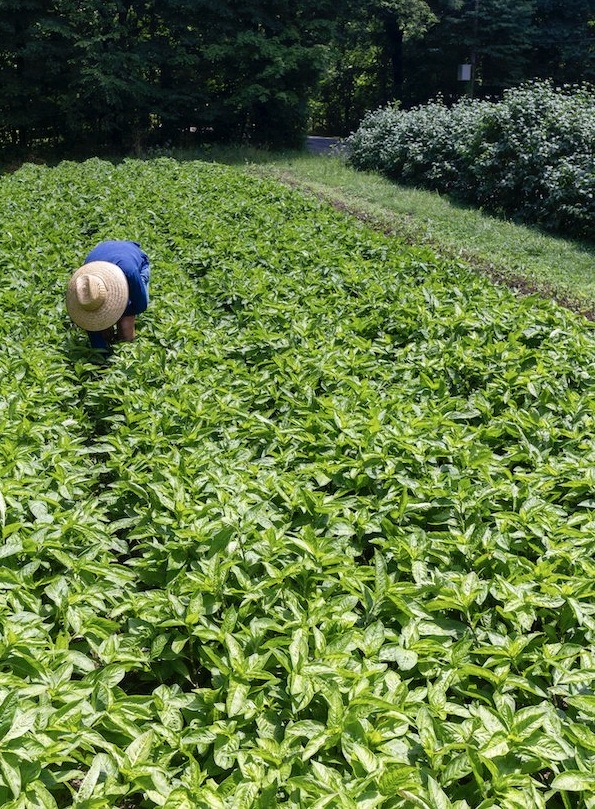This is a detailed color photograph taken outdoors during the day, capturing a lush, green field of ankle-high vegetation arranged in neat rows. In the left middle section of the image, a person is bent over, facing towards us but obscured by a light brown straw hat with a dip in the top, rendering their features invisible. The person is dressed in a long-sleeve blue shirt and blue jean shorts, with their left arm resting on their left knee as they appear to be picking items from the vegetation. To the right, the greenery transitions into darker green bushes, and in the background, there is a wall or possibly a road with dense vegetation and trees growing over it, providing a natural barrier that frames the cultivated field.